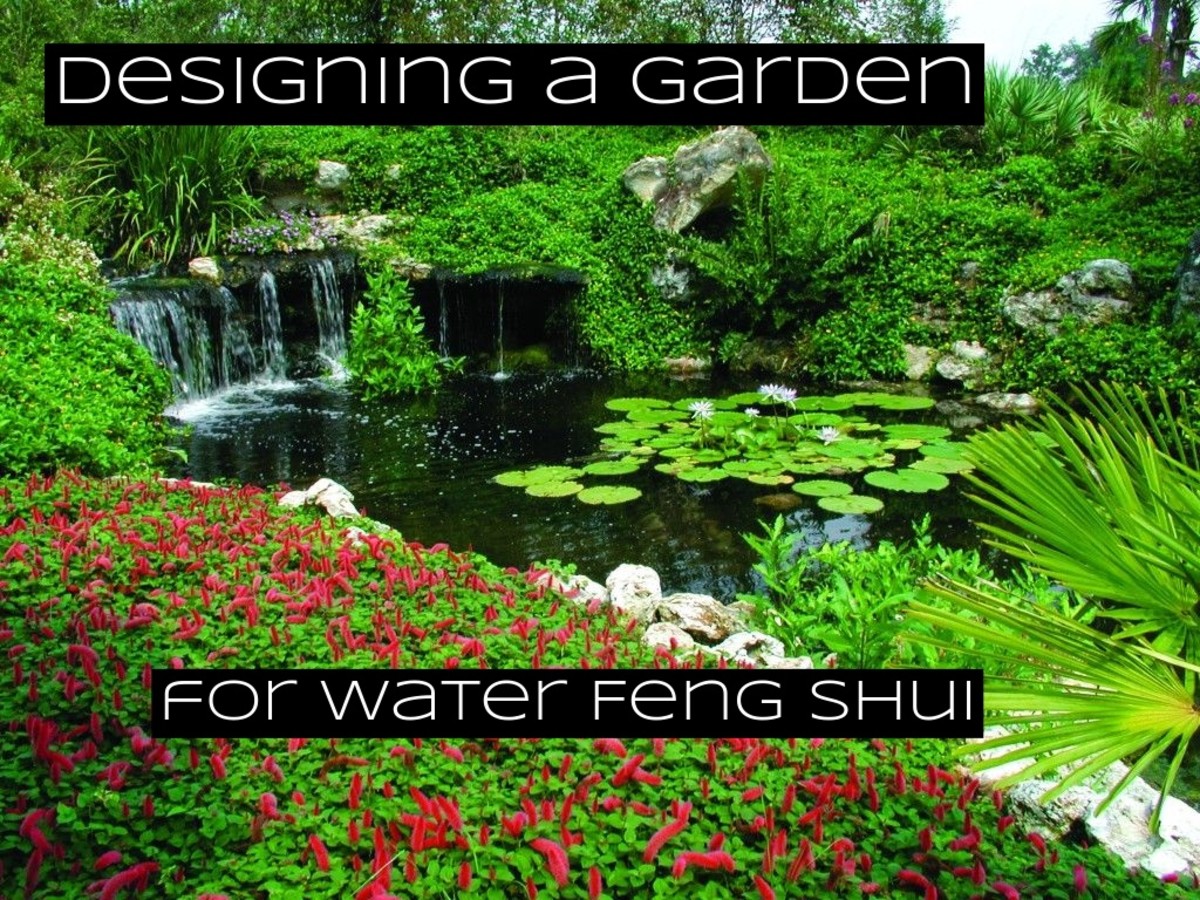This image caption highlights a serene garden designed for water feng shui, prominently featuring a tranquil pond with lush green lily pads. A gentle waterfall feeds into the pond, set amid various shrubs and clusters of greenery. On the bottom left, a burst of pink flowers with verdant leaves adds vibrant color, while in the bottom right, a small palm tree stands tall near a couple of boulders nestled in the grass. Far in the distance, numerous trees contribute to the garden's lush backdrop. The sky above is a soothing blend of blue and white. The garden's design theme is reinforced by text that appears in white font on black rectangles: "Designing a Garden" at the top and "For Water Feng Shui" at the bottom.